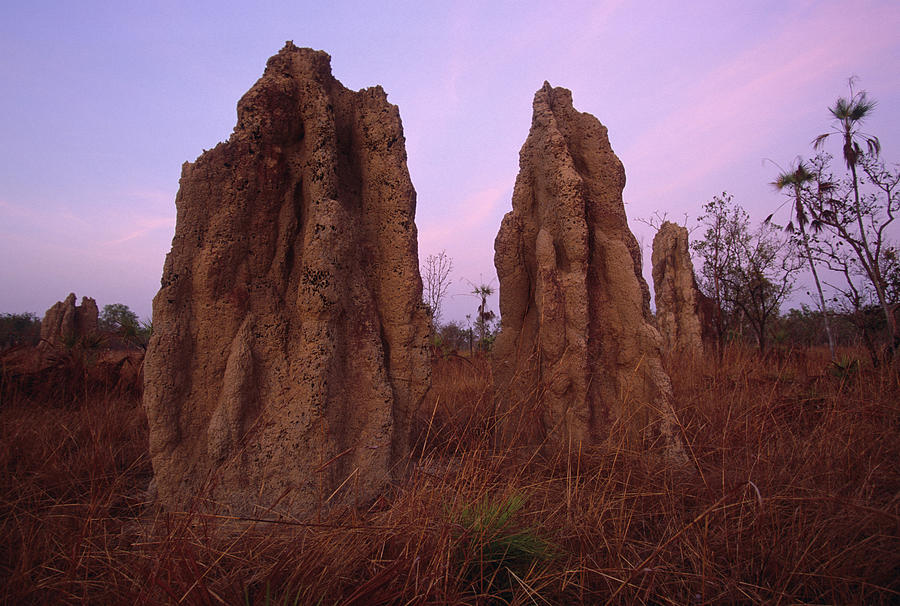The image captures an outdoor scene during sunset, with a sky beautifully blending shades of purple, light lavender, and hints of blue and pink. In the distance on the right-hand side, there are young, bare trees sparsely spread out. The foreground is dominated by overgrown, dried-out grass, resembling hay in some parts. Amongst the grass stand three jagged, mud-like rock formations, resembling termite mounds, arranged with one rock on the left and two on the right—one closer to the viewer and the other further back. The landscape has a slight haze, adding a soft, dreamy quality to the scene.